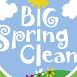This very small, square image, reminiscent of a thumbnail, features a light blue background imitating a cartoonish sky. Across the entire image, it reads "Big Spring Clean" in big, whimsical white letters, with curling S's, P's, and G's. The "I" in "Big" is dotted with a bright, cartoonish sun. Flanking the word "Big" are two puffy white clouds. Below "Clean," there's a small green hill adorned with a few colorful daisies in pink, yellow, and white. The overall aesthetic is cheerful and childlike, exuding a playful, happy vibe.